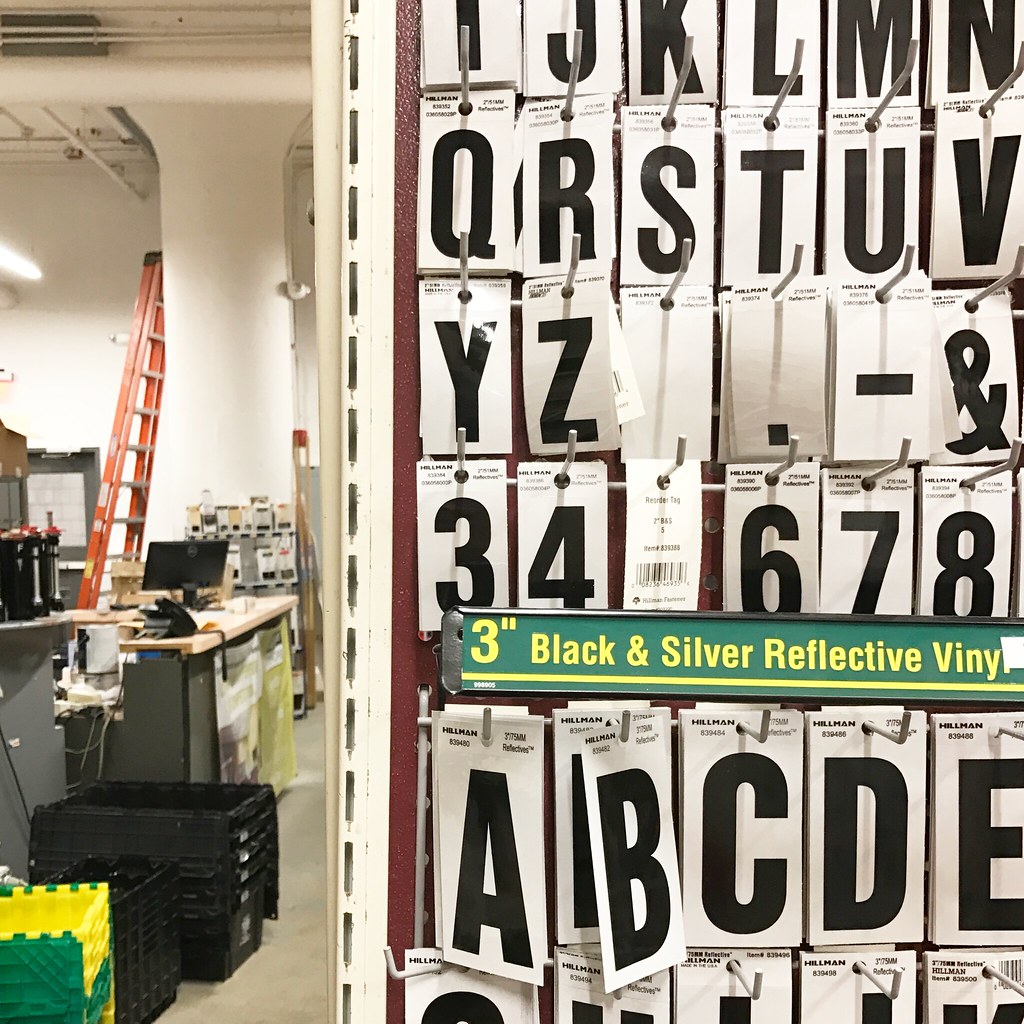This is an image taken inside what appears to be a store, possibly a hardware store. Dominating the right two-thirds of the image is a white metal stand displaying various rectangular letter and number stickers for sale. The stand's banner reads "3-inch black and silver reflective vinyl" in prominent yellow text, indicating these are reflective vinyl stickers. 

The letters and numbers are arranged in a somewhat organized fashion, with larger letters A, B, C, D, and E at the bottom. Above these, in ascending rows, smaller characters can be seen, starting with I, J, K, L, M, N at the top, followed by Q, R, S, T, U, V, and then Y, Z, with symbols like a period, dash, and ampersand sprinkled among them. Numbers 3, 4, 6, 7, and 8 are also visible.

To the left of the sticker display stands a large white pillar against which a tall red stepladder is leaning. Adjacent to this pillar, there are green, yellow, and black plastic totes, some of them appearing to be storage containers. A gray and beige counter holds a computer monitor, and additional shelves are seen in the background, suggesting the presence of more tools or merchandise.